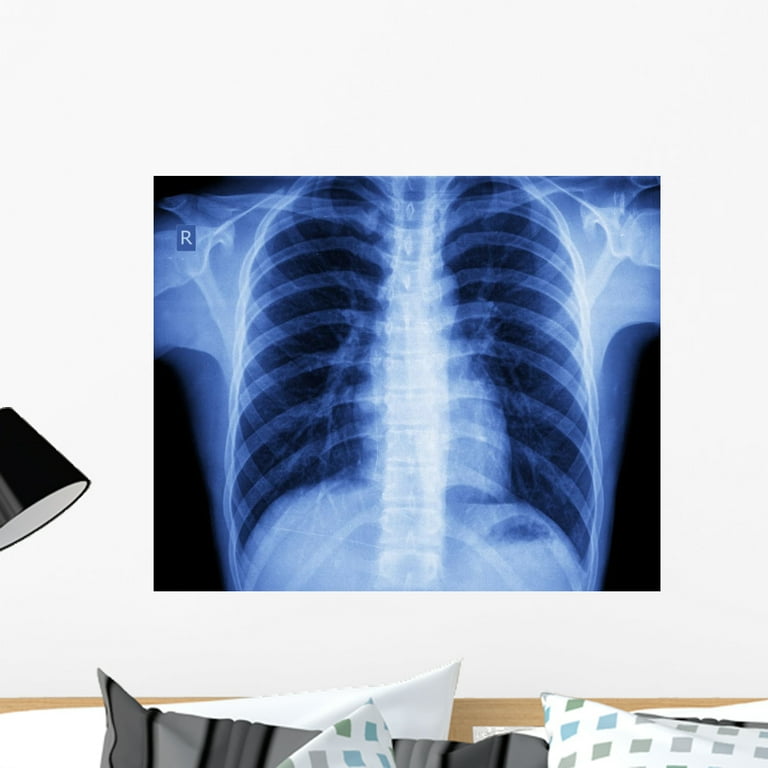The image portrays a digital reproduction of a chest x-ray, showcasing ribs, spine, shoulders, and a faint outline of the heart, all rendered in a standard blue tinge characteristic of x-ray imagery. This x-ray is used as a poster or canvas art, hung prominently on a wall above a piece of furniture. This furniture, likely a bed or couch given the presence of pillows and a brown backboard, anchors the scene. The x-ray also features a faint character-like mark at the top left corner, resembling a watermark. The overall composition blends the x-ray's clinical appearance with a home setting, creating a unique and unconventional piece of decor with contrasting elements.